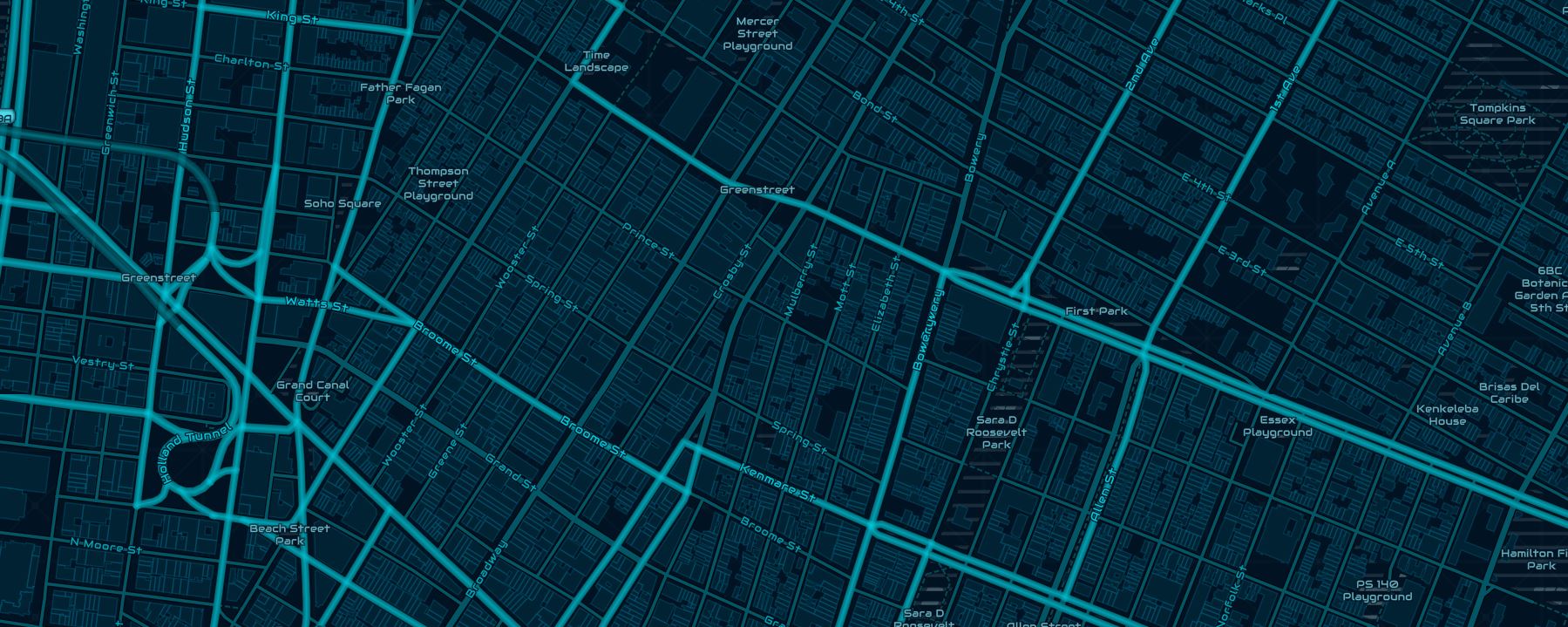This image showcases a detailed street map of New York City, characterized by a predominantly greenish-blue hue that lends a modern, clean aesthetic typical of sat-nav visuals. The major thoroughfares are highlighted in a lighter greenish-blue color, standing out with their thicker, more prominent lines, while the minor roads are depicted as darker, thinner pathways. The map subtly outlines the buildings in a darker shade, adding depth without overwhelming detail. Central to the composition is Sarah D. Roosevelt Park, serving as the focal point amidst the urban grid. The map is rectangular in shape and offers a clear, high-contrast visual experience, enhanced by the aquamarine and light bluish-green tones against a black background. Designed with a minimalist touch, it provides essential information by naming only the main streets, making it both functional and visually appealing.